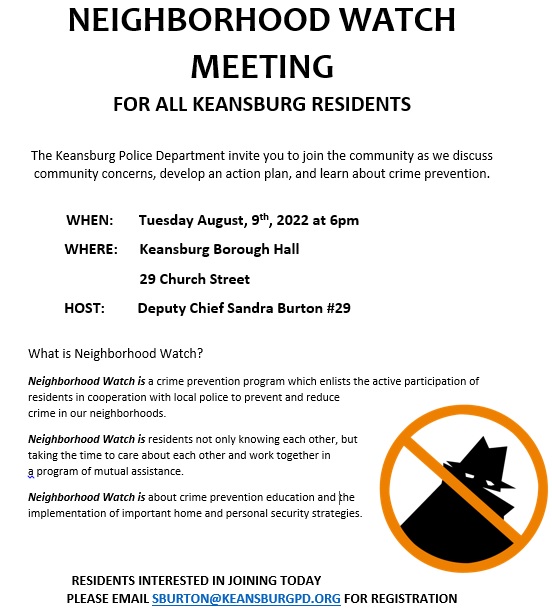The image is a digital flyer on a white background with primarily dark text, announcing a "Neighborhood Watch Meeting for All Keensburg Residents." The main text is in large black font, with a subheading in smaller black font that states: "The Keensburg Police Department invites you to join the community as we discuss community concerns, develop an action plan, and learn about crime prevention." The flyer details the event as taking place on Tuesday, August 9th, 2022, at 6 p.m. at Keensburg Borough Hall, hosted by Deputy Chief Sandra Burton. It additionally explains that Neighborhood Watch is a crime prevention program that involves residents cooperating with local police to prevent and reduce crime, emphasizing community collaboration and education on crime prevention. There is also an illustration featuring the silhouette of a thief within a green circle crossed out with a diagonal line, symbolizing "no crime." For those interested in joining, the flyer provides registration information via an email address: sBurton@KeensburyPD.org.